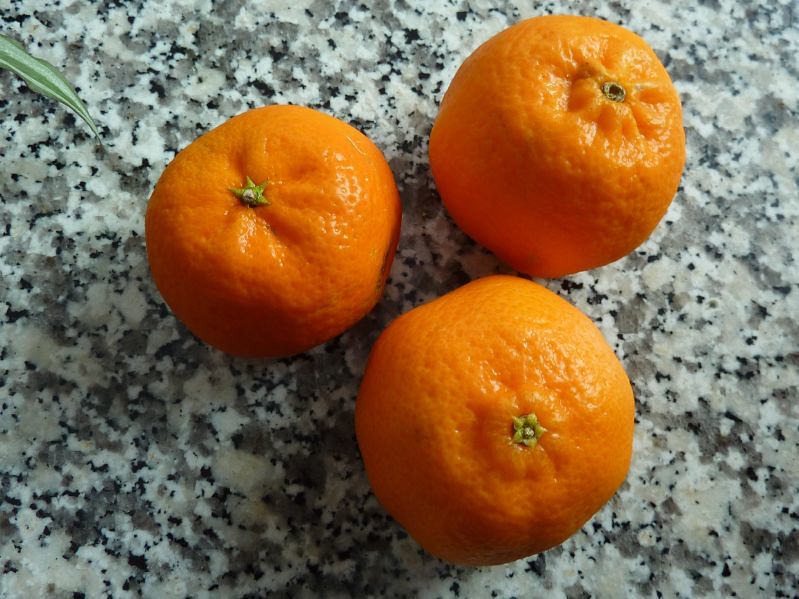The photograph captures an inviting arrangement of three vibrant, bright orange fruits—likely tangerines, tangelos, or Mandarin oranges—resting on a richly textured marble countertop that blends hues of brown, black, and white. The fruits are positioned in a triangular formation, with one at the top left, one at the top right, and one at the bottom, filling much of the frame and casting subtle shadows from a light source. In the top left corner of the image, a dark and lighter green leaf peeks into the frame, adding a touch of natural contrast. The glossy, easy-to-peel appearance of the fruits paired with the contrasting colors of the marble surface creates a vibrant and appetizing visual, making the simple scene of someone’s snack look particularly delectable and inviting.